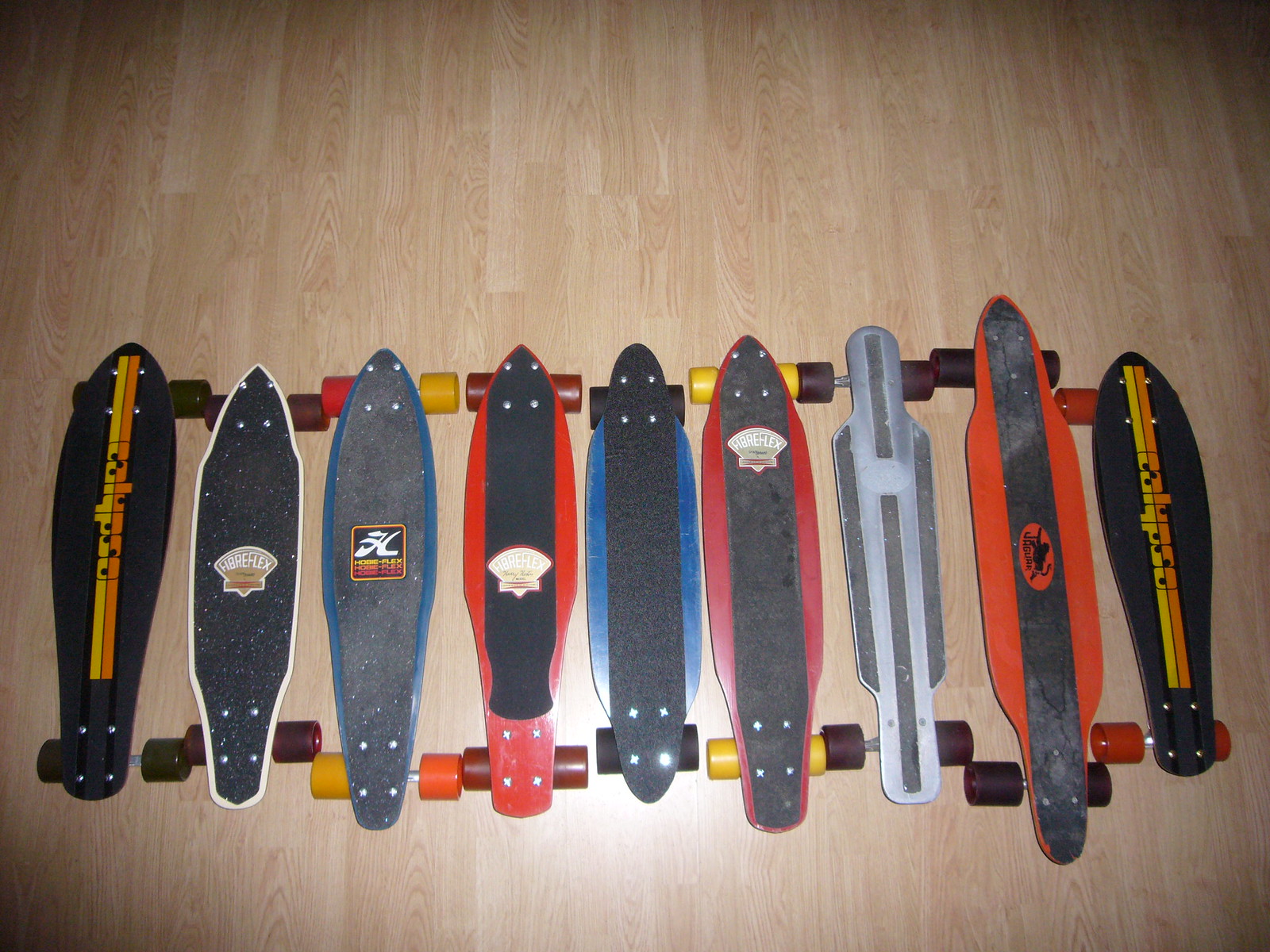This photograph captures an organized row of nine longboards laid out on a light brown hardwood floor, taken from a downward angle inside a home. The boards showcase a variety of colors and designs. Most feature black grip tape at their centers, with bright accents of red, blue, yellow, orange, gray, and silver on their edges. Distinctively, these longboards are not of the typical skateboard shape but have unique contours and ends, emphasizing their varied designs. The wheels are positioned outside the edges, making them visible. Some boards display logos and insignias, although they are not clearly discernible. The light in the room highlights the array of colors, reflecting on the grip tape and the scuff marks, indicating use.